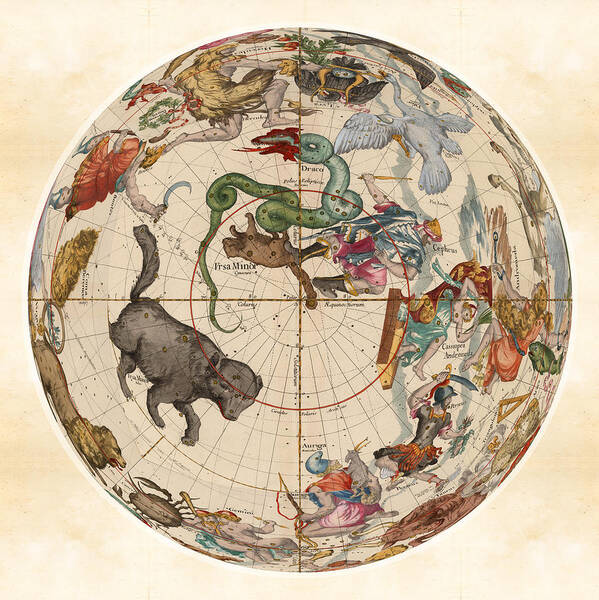This image depicts a detailed map of constellations, centred around a brown cross that divides it into four quadrants, all set against a marbled pink and yellow background. The circular map features various mythical and real animals, as well as human figures, each representing different constellations. Prominent figures include Ursa Minor, shown as an upside-down bear, a grey ferret, and a snake emitting fire located on the lower left. On the right side, a griffon can be seen in the upper quadrant. Additional characters include a large white bird, a goat hanging from the back of a blue-hatted warrior with a bow and arrow, and another warrior sitting on a sled, armed with a sword. Human and humanoid figures are scattered across the map, with one holding a rifle and another wielding a scimitar. Constellations such as Cancer, the crab, add to the celestial theme of this highly intricate representation of the sky.